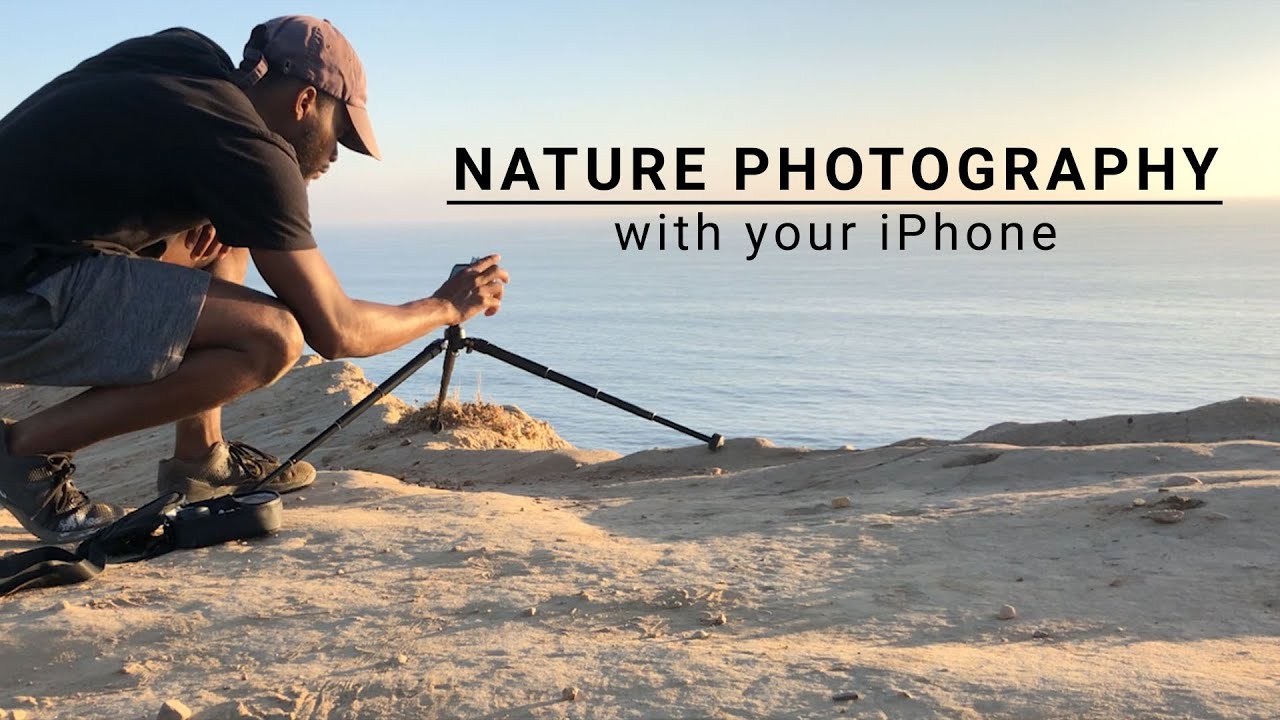This color photograph captures a young black man kneeling down on a dusty cliff surface above a large body of water, possibly the ocean, during a golden light period near sunset or sunrise. He is setting up his mobile phone on a wide-legged tripod. The man is dressed in a dark-colored t-shirt, gray shorts, a brown baseball cap, and dark low-cut sneakers. Beside him, there is a black case on the ground. Superimposed in the upper right portion of the image is a bold black title that reads "Nature Photography with your iPhone." The scene showcases the vast expanse of water meeting the horizon under a blue sky, accented by the warm golden light.